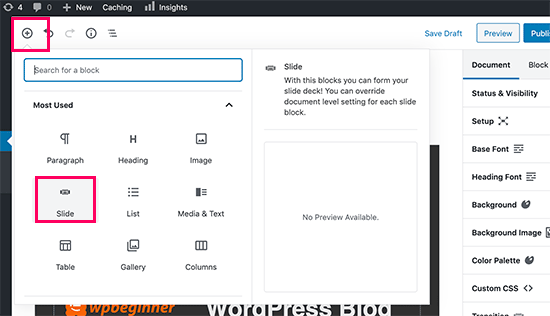The image is a detailed screenshot of a blog customization interface, designed to guide users through adjusting their settings before publishing. 

At the top of the interface, there is a black circular button with a plus sign inside, highlighted by a red square around it. Next to this button are two arrows for navigating: a left-pointing arrow and a right-pointing arrow that is grayed out, indicating it's currently inactive. Further along, there is an information icon (a circle with the letter "I" inside) followed by four horizontal lines, suggesting a menu.

On the opposite side of this top bar, there are three blue buttons labeled "Save Draft," "Preview," and "Publish." Below this header, there are tabs for "Document" and "Block" settings. Within these tabs, users can configure various options including "Status and Visibility," "Setup," "Base Font," "Heading Font," "Background," "Background Image," "Color Palette," and "Custom CSS."

The central area of the page prominently features a blue box with the text "Search for a block" and a section labeled "Most Used." Icons in this section represent different content blocks such as Paragraph, Heading, Image, Slide, List, Media & Text, Table, Gallery, and Columns. The "Slide" block is marked with an additional red box around it, drawing attention to it.

Accompanying these blocks, there is explanatory text stating, "With these blocks, you can form your slide deck. You can override document-level settings for each slide block." Below this text, there's a gray box indicating "No preview available."

At the bottom of the page is a black footer bar containing white text that reads "WordPress blog." Next to it are the letters "W P O E G I N N E R" leading into "WP beginner" in orange letters.

This detailed caption outlines the image's elements, making it easier to understand the blog customization process.